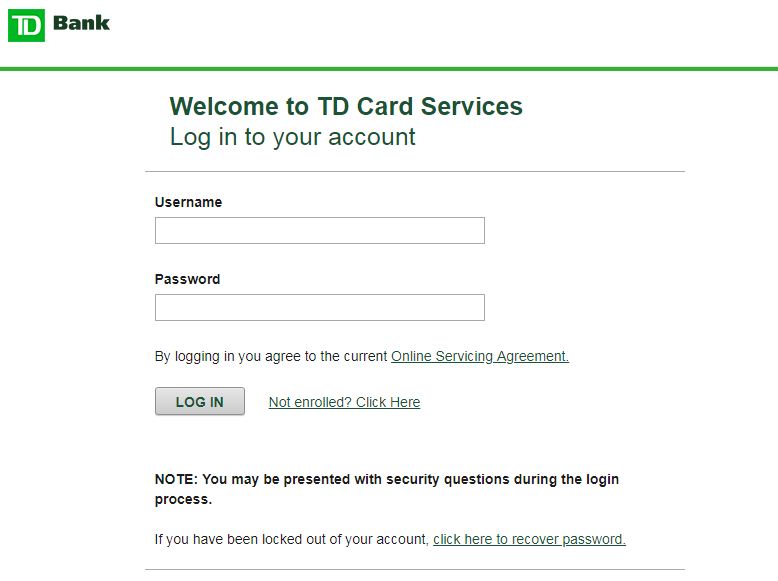This is a detailed description of a TD Bank login webpage:

The TD Bank login webpage prominently features the TD Bank logo, characterized by its familiar green background with white lettering—'TD' in white and 'Bank' in black positioned to the right. Below the logo, a green horizontal line sets off the sections of the page.

The headline "Welcome to TD Services" is displayed in bold, dark green letters, providing a welcoming prompt to users. Directly beneath this header, in lighter green text, is the instruction "Log into your account." Underneath this, a black horizontal line separates the header from the login fields.

The first field labeled "Username" appears in dark black letters, accompanied by a section for users to enter their username. Below this, the "Password" field is also marked in dark black text, with a corresponding input section.

A note then states, "By logging in, you agree to the current Online Service Agreement," reinforcing the terms of service. Following this disclaimer, a green "Log In" button is provided for users to access their accounts.

Further down, the page informs users that they may be presented with security questions during the login process and offers a link, "If you have been locked out of your account, click here" in green, for account recovery options. This notification concludes with a faint black line.

Overall, the page is designed to be straightforward, clearly guiding TD Bank account holders through the login process with minimal distractions.